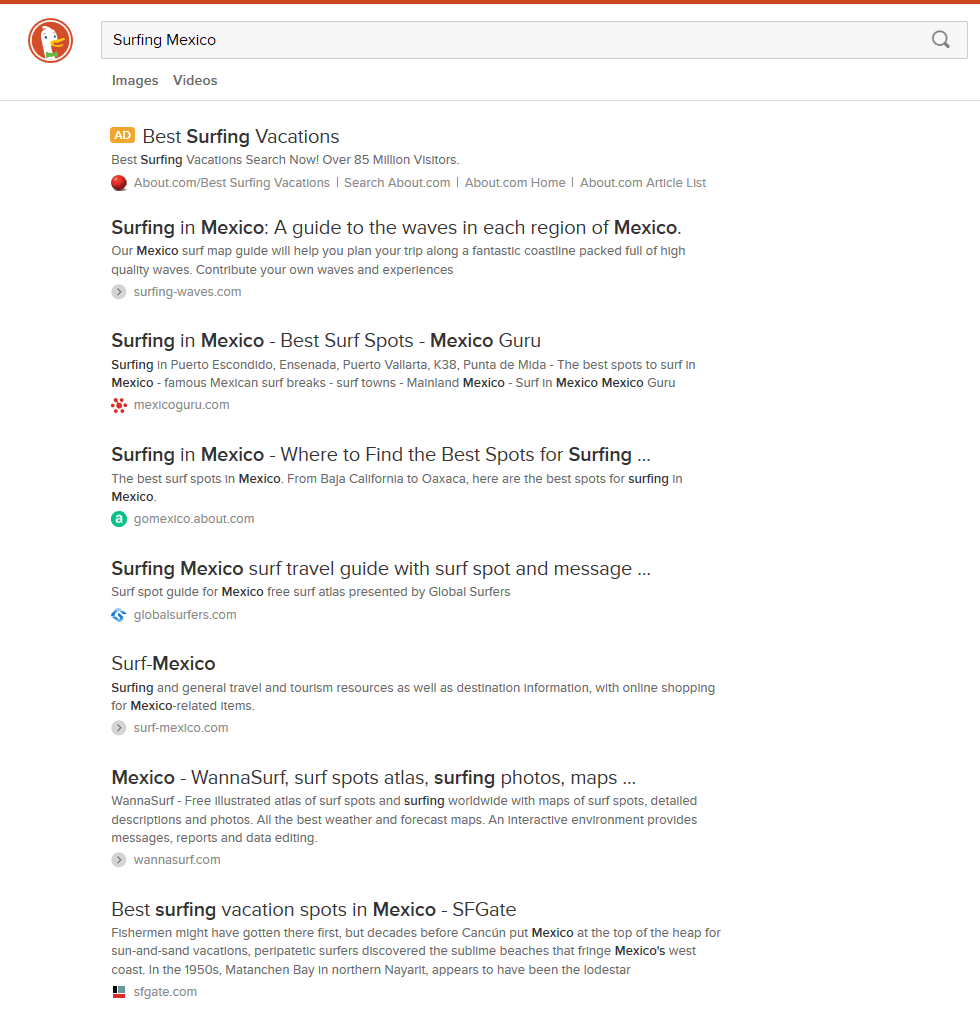The image appears to be a screenshot of search results from the DuckDuckGo search engine. At the top of the image is a prominent red line that spans the entire width. Directly below this is the recognizable DuckDuckGo logo, accompanied by a search field containing the query "Surfing Mexico." To the right of this search field is a search icon in the form of a magnifying glass.

Below the search bar, there are options for filtering results by images and videos, separated by a thin gray line that extends across the width of the screen. The first search result is an advertisement, distinguishable by its yellow ad highlight, titled "Best Surfing Vacations," which includes additional details. 

Further down, the organic search results begin, starting with:
1. "Surfing in Mexico: A Guide to the Waves in Each Region of Mexico" - offering comprehensive information on surf spots across the country.
2. Another link, "Surfing in Mexico: Best Surf Spots, Mexico Guru" - which provides insights into the top surfing locations.
3. "Surfing in Mexico: Where to Find the Best Spots for Surfing" - detailing various surf destinations.
4. "Surfing Mexico: Surf Travel Guide with Surf Spot and Massage" - featuring a blend of surfing and relaxation tips.
5. "Surf Mexico" - likely a general overview or additional resources related to surfing in Mexico.
6. "Mexico: Want to Surf? Surf Spots, Atlas, Surfing Photos, Maps" - a link offering an extensive guide with visual aids.
7. "Best Surfing Vacation Spots in Mexico - SF Gate" - highlighting prime locations for surf vacations.

Each result includes a hyperlink and a concise description, all set against a clean and minimalistic white background, making the information easy to read and navigate.